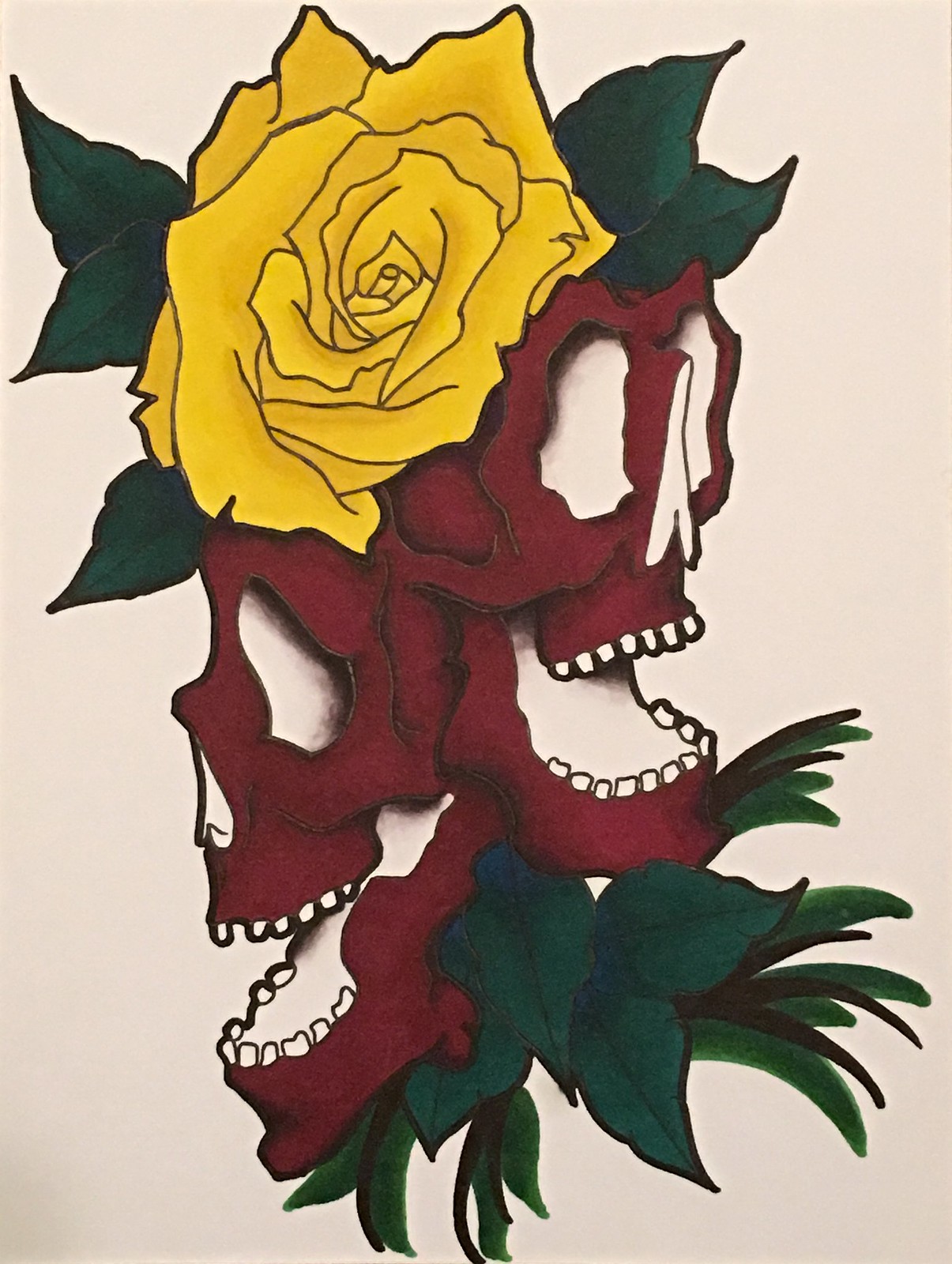The image depicts a vibrant and artistic rendition of a yellow rose perched atop two dark red skulls. The yellow rose, complete with green, pointy leaves and stylized petals, sits prominently above the skulls, capturing immediate attention with its vivid coloration. Below the rose, the two skulls are fused back-to-back, facing away from each other with their large, expressive eyes and wide, tooth-lined mouths open in a seemingly excited or smiling manner. The skulls are deep red or maroon in color, with striking white gaps in their eyes, noses, and mouths, emphasizing their bone-like features. Surrounding and beneath the skulls are more green, pointy leaves and blades of grass, varying from dark to light green and black, integrating the skulls into the plant-like composition. The overall effect is a colorful, stylized, and slightly cartoony image that merges the macabre with the botanical, creating an intriguing and visually captivating scene.